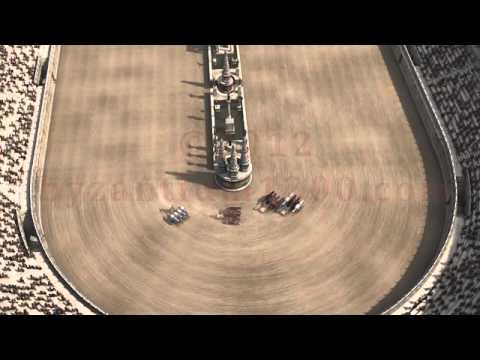This image resembles a movie scene or an old documentary clip, featuring a U-shaped segment of an elliptical racetrack, which appears to be crafted from dirt or sand, showcasing a light beige hue. The track is populated by what seems to be four groups of indistinct, blurry figures that could be horses, chariots, or similar racing apparatuses, racing around the bend. The aesthetic of the track and surrounding structures evoke a futuristic, almost Star Wars-like design. Central to the image, amidst the track, are unique tower-like structures, enhancing its enigmatic vibe. Encircling the track are spectator stands, comprised of large, stone steps, sparsely dotted with black figures that are presumably people, blurred in the aerial, downwards perspective of the image. Overall, the details are somewhat unclear, lending an air of mystique to the scene.